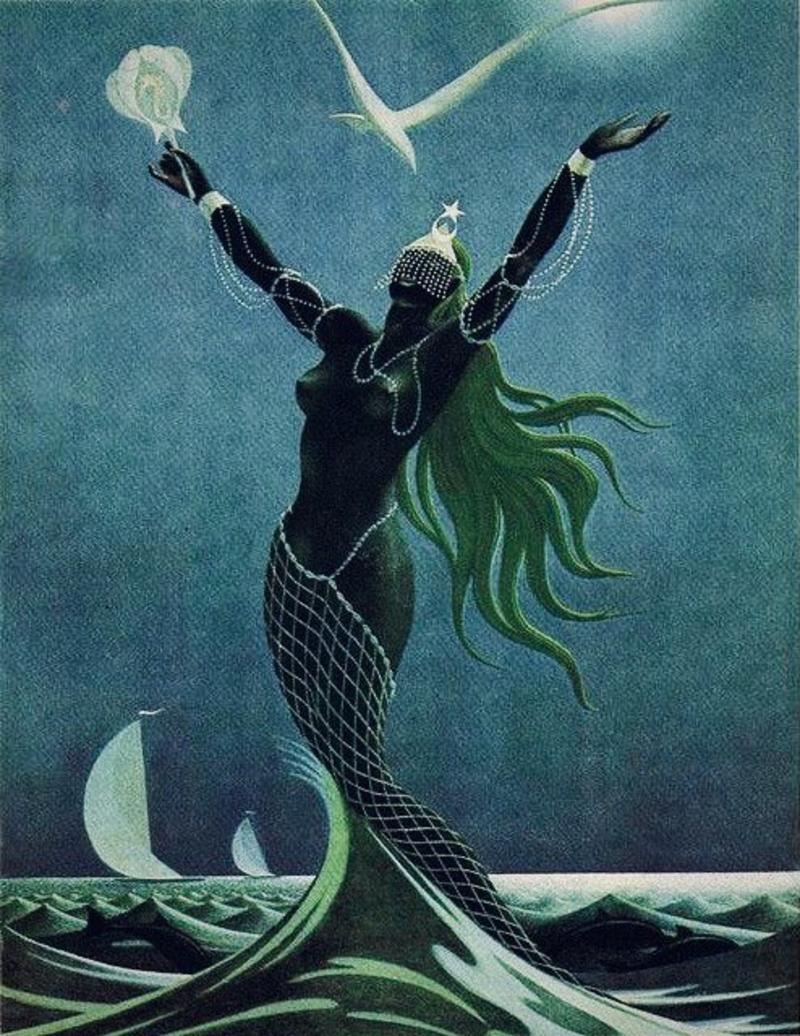This captivating Art Deco-style image features a striking black mermaid emerging from the sea, set against a rich teal, dark bluish-green background. The central figure, adorned with flowing green hair, stretches her arms towards the heavens, holding an enigmatic object in her right hand. She is bedecked in elaborate pearl jewelry: bracelets and necklaces that extend gracefully from her wrists to her elbows and upper arms. She appears topless, with her lower half seamlessly transitioning into a fishnet-like skirt decorated with pearls, which elegantly drapes from her right hip down to her concealed tail in the water. A tiara adorned with a moon and star crowns her head, with a veil of pearls cascading over her face, partially obscuring her features. Above her, a stylized white seagull can be seen, while the barely visible moon glows in the top right corner. The sea below her is depicted with stylized waves in light and dark green, accented with touches of white and black, and two stylized yachts appear in the bottom left quadrant of the image. This evocative scene, rich in oceanic hues and intricate details, speaks to a fantastical, stylized vision, reminiscent of comic book art.